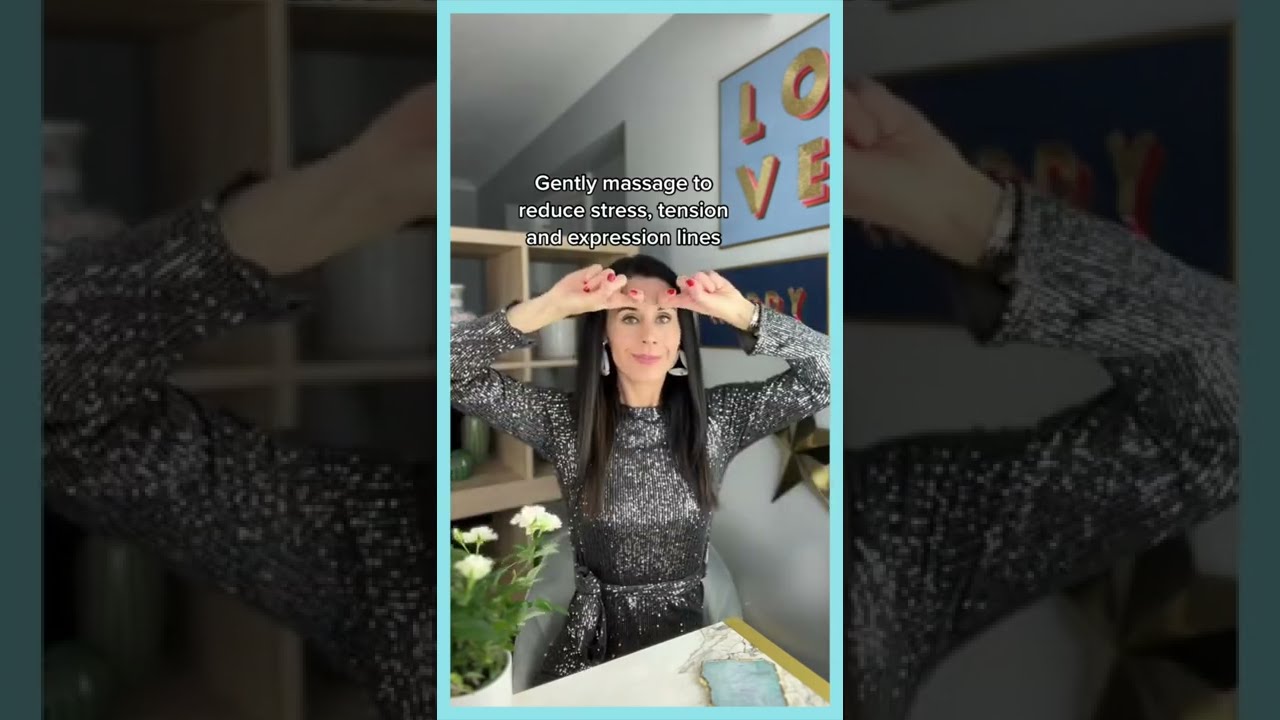In the image, a woman with long black hair and a light complexion is dressed in a glittery, long-sleeved sequined dress in either gold or black. She is seated and smiling, performing a forehead massage as instructed by the text overlay that reads, "Gently massage to reduce stress, tension, and expression lines." This text is in white font and positioned above her. The woman's hands are bent at the elbows, with her fingers resting on her forehead. She is adorned with large, hanging earrings and is wearing red nail polish. The background features a room with white walls, some shelving, and a framed sign that spells "LOVE" in gold letters on a blue background. Additionally, the image composition includes two magnified, slightly blurred sections: one focusing on her hand on her forehead and the other on her arm. To the side, there's probably additional wall art and a plant with white flowers.